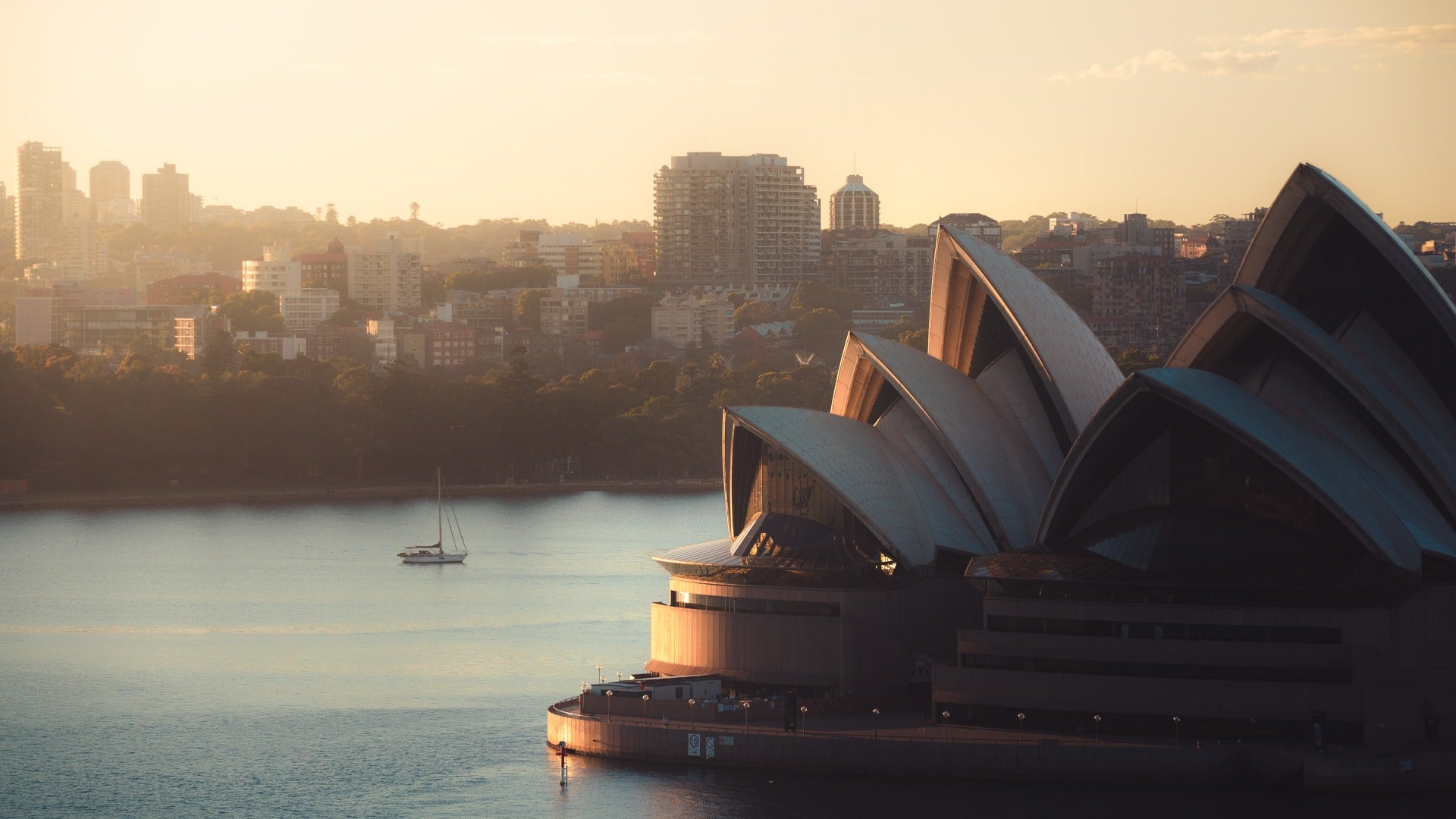The image captures the iconic Sydney Opera House, majestically situated on a peninsula in Sydney Harbour, Australia. The unique architectural design of the Opera House features three prominent, white, pointed shell-like structures that resemble rounded triangles layered in two columns. Known locally as resembling "nuns in a scrum," these roofs make the building instantly recognizable. 

To the left of the Opera House lies the expansive, blue waters of the harbour, within which a private sailboat floats. Beyond the water, the shore reveals a dense skyline of buildings that are part of the bustling city of Sydney. The scene appears to be set during either sunrise or sunset, as the entire landscape is bathed in a serene, orange glow, adding warmth to the otherwise gray sky scattered with white clouds. The presence of such distinguished landmarks against the backdrop of an awakening or resting city encapsulates the harmonious blend of natural and urban beauty.